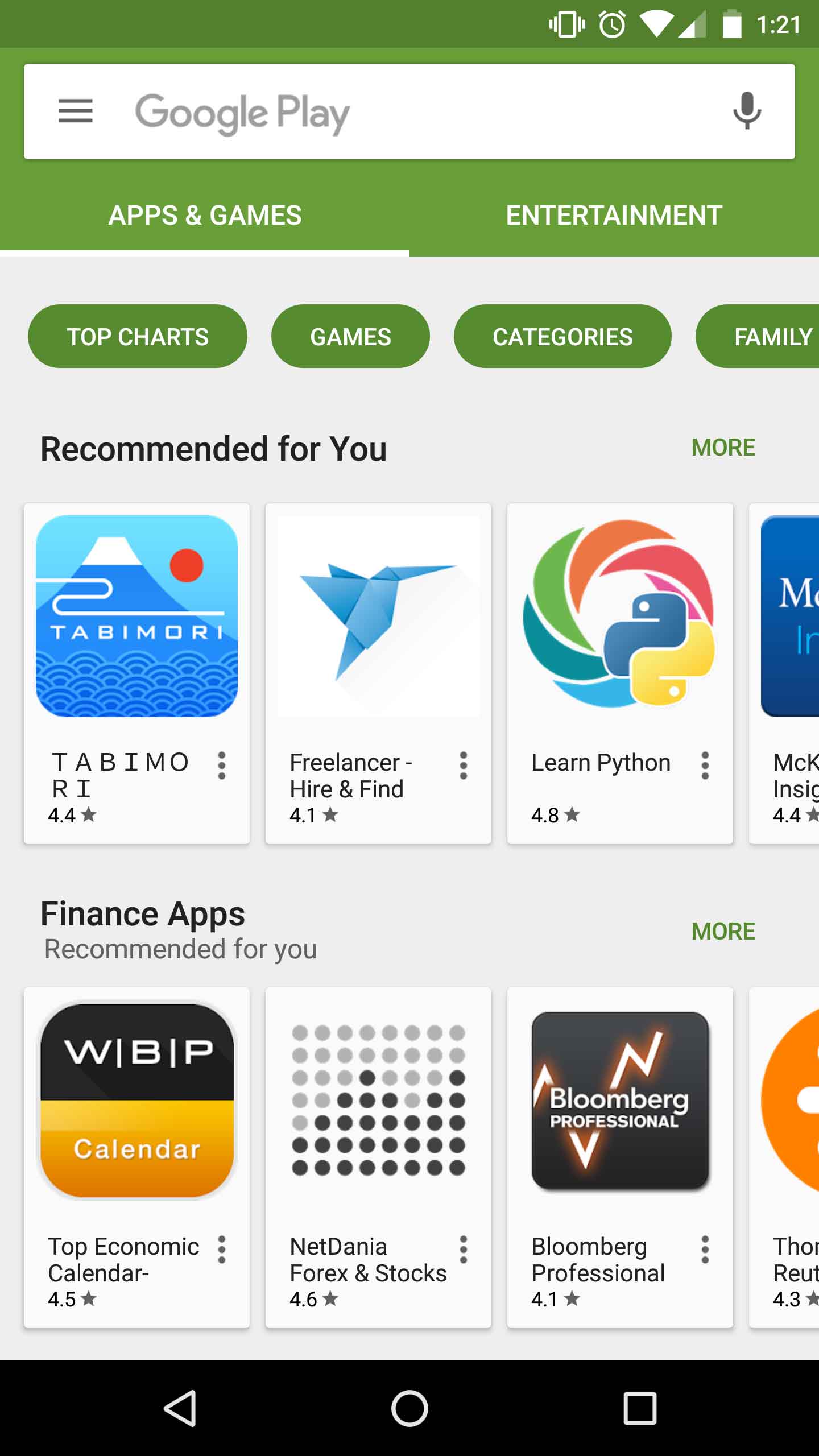The image displayed on someone's cell phone screen shows a nearly full battery and a time reading of 1:21. The connection signal is very strong. At the top of the screen, there's an icon resembling a watch alongside the time. The Google Play app is open with "Google Play" typed in the search bar. A microphone icon is visible, indicating that voice search is an option.

In the Google Play interface, the user has navigated to the "Apps & Games" section, highlighted in green, grouped under various categories like "Top Charts," "Games," "Categories," and "Family." "Recommended for You" is prominently displayed, with suggestions including:

1. "Tab Emo Freelancer Hire and Find"
2. "Learn Python WBP"
3. "Calendar Daniel"
4. "Forex and Stocks"
5. "Bloomberg Professional"

The other recommendations are partially cut off on the right side of the screen, making only portions of subsequent app titles visible. Each app recommendation is presented within oblong green bars.